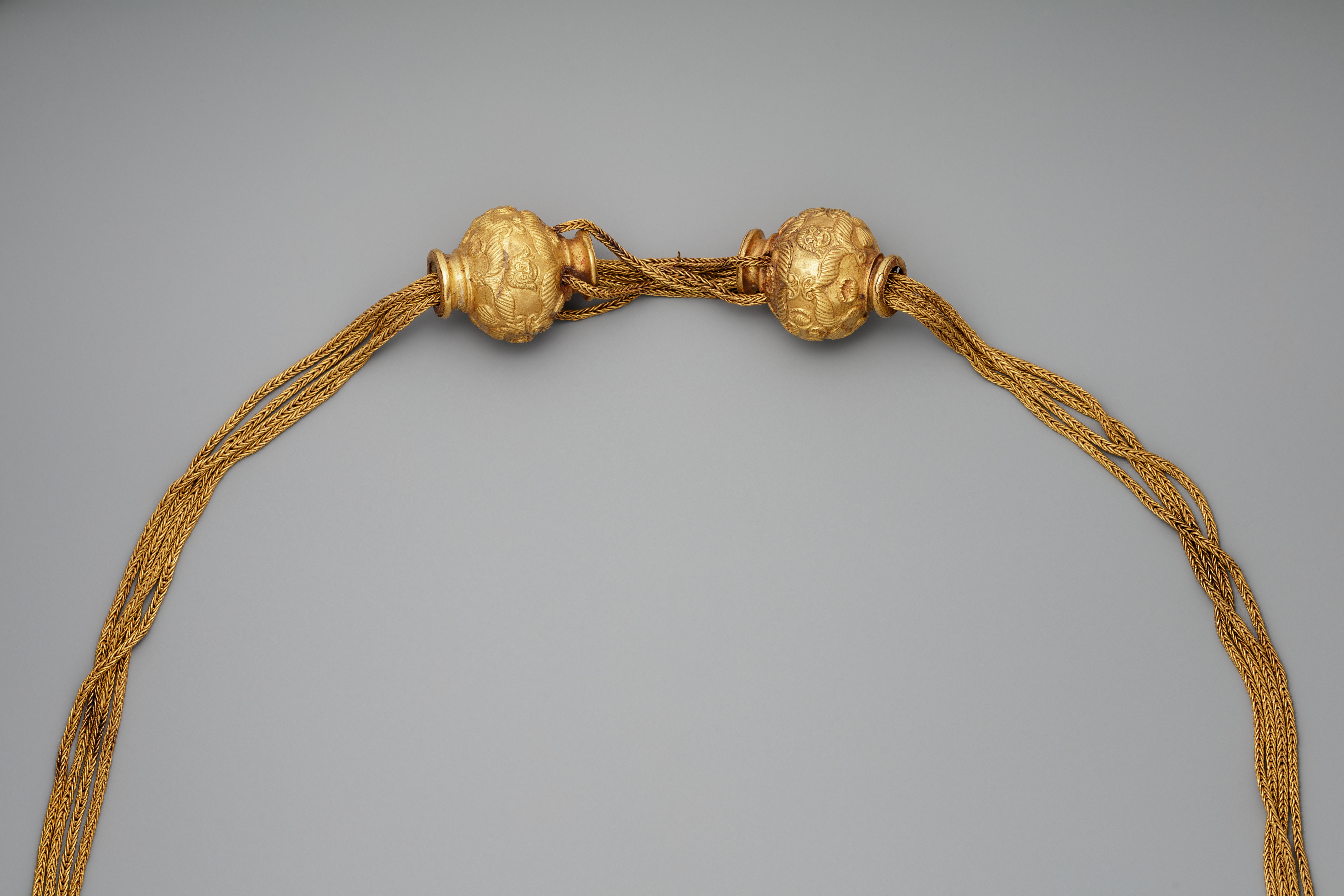The image showcases a section of a gold-colored necklace set against a light gray background. The necklace features two intricately designed, golden goblet-like components, positioned about an inch apart near the top of the image. These goblet components are adorned with detailed patterns that include what appear to be monkey faces and other animals. The necklace comprises multiple strands, possibly four, in a herringbone style, interwoven through the openings in the goblet pieces. The strands drape down and blend into the gray background. The overall aesthetic of the image leans towards a gold-themed design, with the exact material of the necklace strands appearing to be a hard metal, although this is not entirely clear from the image.